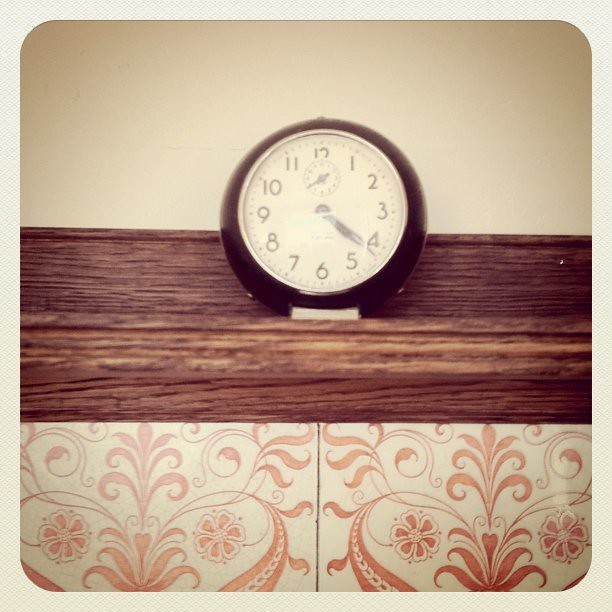This vintage photograph, characterized by its rounded corners and yellowed mat, exudes an antique charm accentuated by the yellow filter tone typical of old images. The scene captures an off-white wall adorned with wallpaper featuring a whimsical, flowy heart design on its lower half. Positioned against this wall is a piece of dark wood furniture, which could be a shelf or a cabinet. Atop this furniture sits a prominent, intricately designed clock with a rounded black exterior and a white base. The clock face includes an additional smaller face nested within it, adding to its unique and intricate appearance.